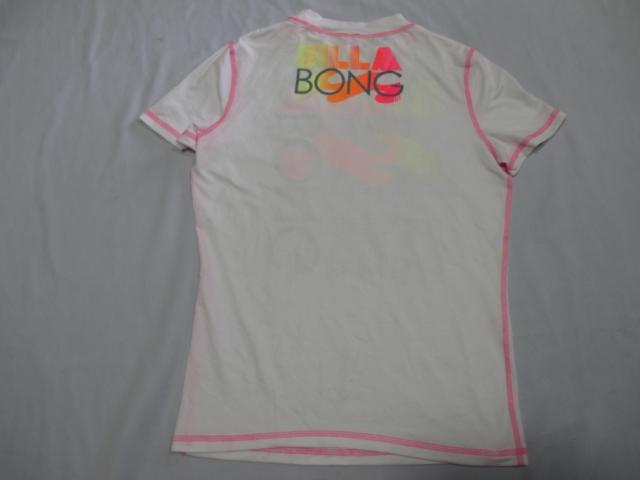The photograph showcases a white short-sleeve t-shirt laid out neatly on a wrinkled white cloth background, providing a textured contrast. The t-shirt features bright pink banding along the seams, neckline, sleeves, and bottom hem, creating a vivid accent against the white fabric. The high neckline shirt displays the brand name "BILLABONG" prominently across the chest. The letters B-I-L-L-A are individually colored, starting with a neon yellow B, followed by orange I, L, L, and finally a pink A. Underneath, the word "BONG" is printed in bold black capital letters, each letter overlayed with a corresponding marker smear – yellow over the B, orange over the O and the N, and pink over the G. The detailed stitching and colorful text give the shirt a vibrant appearance. Additionally, the back of the shirt is slightly see-through, revealing another instance of the brand name "BILLABONG." The t-shirt is centered in the image, with the entirety of its design fully visible against the white background.